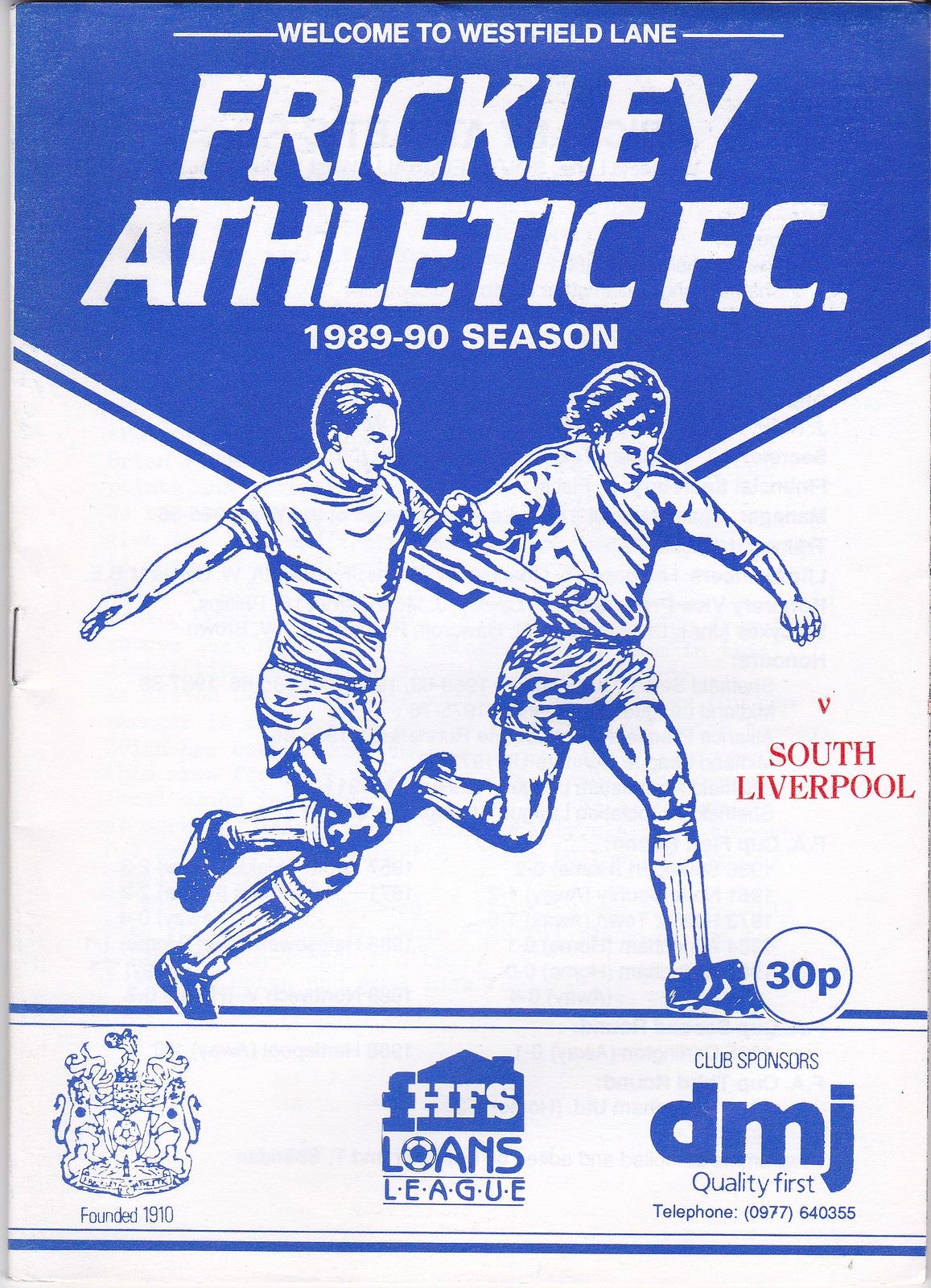The program cover for the 1989-90 season of Frickley Athletic F.C., set against a blue and white backdrop, prominently features the heading "Welcome to Westfield Lane" with horizontal lines extending from either side. Below this, in larger white text, is the name "Frickley Athletic F.C." followed by the season designation. A central animation, rendered in blue and white, depicts two male soccer players in motion—one with short hair and a straightforward athletic outfit, and the other with longer, shaggy hair. The front player, poised to kick a soccer ball that is actually labeled "30P", extends his arms with one crossing in front of the other player. Red text reading "Vs. South Liverpool" is positioned beneath his hand. At the bottom, three emblems are lined up, detailing crucial information: the leftmost emblem denotes "Founded 1910" with two lions and flags, the central emblem is for the "HFS Loans League" featuring a blue house background, and the rightmost emblem indicates the club sponsor "DMJ Quality First" along with a contact telephone number.